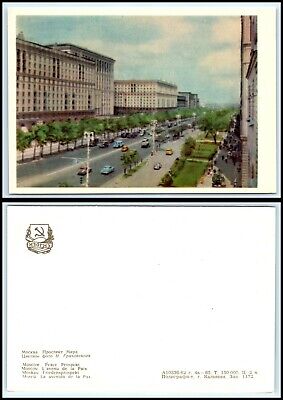The image depicts both the front and back of an old-fashioned postcard, potentially originating from the Soviet Union. The front showcases a faded painting of a small town or cityscape with a distinctly aged appearance, featuring green, off-blue, light blue, white, black, and gray hues. The scene captures a street lined with two to three-story buildings, long with many windows, trees, and significant road traffic featuring Soviet-style utility cars. The angle suggests it was taken from the second story of a building, looking across the street. The sun is positioned in the middle of the sky, illuminating the quaint, bustling urban environment.

On the back of the postcard, a small hammer and sickle emblem is visible in the upper left corner, indicative of its Soviet origin. The rest of the space is predominantly blank white, with some text that is too small and blurry to decipher, possibly in Cyrillic. Although there are similarities to a QSL card, typically used by ham radio enthusiasts, the postcard lacks specific stamps or definitive markings for such a purpose, reinforcing its identity as a vintage postcard potentially available for purchase in a store decades ago.